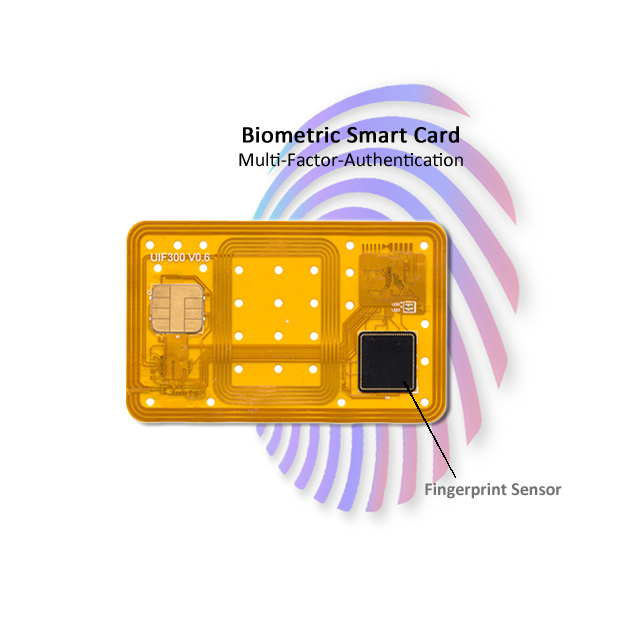The image is an advertisement for a cutting-edge biometric smart card featuring multi-factor authentication. At the top center, bold black text reads "Biometric Smart Card Multi-Factor Authentication." The backdrop of the image showcases an artistic representation of a fingerprint in soothing pastel shades of blue, purple, and pink. Dominating the center of the image is a yellow, credit card-shaped device embellished with white polka dots and intricate line designs. The card prominently displays the text "UIF 300 VO.6" at the top left. Intricately detailed, the card integrates a chip on its left side, symbolizing conventional smart card functionality. Highlighted in the bottom right corner of the card is a small black square, clearly labeled as the fingerprint sensor. Transparent arrows point to the sensor, emphasizing its role in the enhanced security features of this innovative smart card.